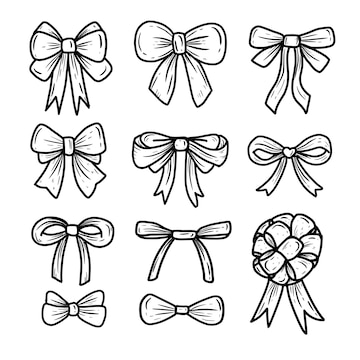This black and white pictorial showcases 11 different ribbon-tying methods arranged in four lines. Each method produces varied styles of bows, ranging from traditional bows with ribbons hanging down to more intricate designs. On the left, the first bow features three loops at different angles with ribbons hanging from the center. Beside it, another bow resembles a classic bow tie with a couple of ends at the bottom. Further, there's a design similar to a hair ribbon that girls often wear, with two long ribbons flowing downwards. The bottom right corner presents a more elaborate, multi-looped ribbon akin to a prize ribbon or a decorative bow you might see on a special gift. This detailed arrangement emphasizes the versatility and aesthetic appeal of ribbon-tying techniques.